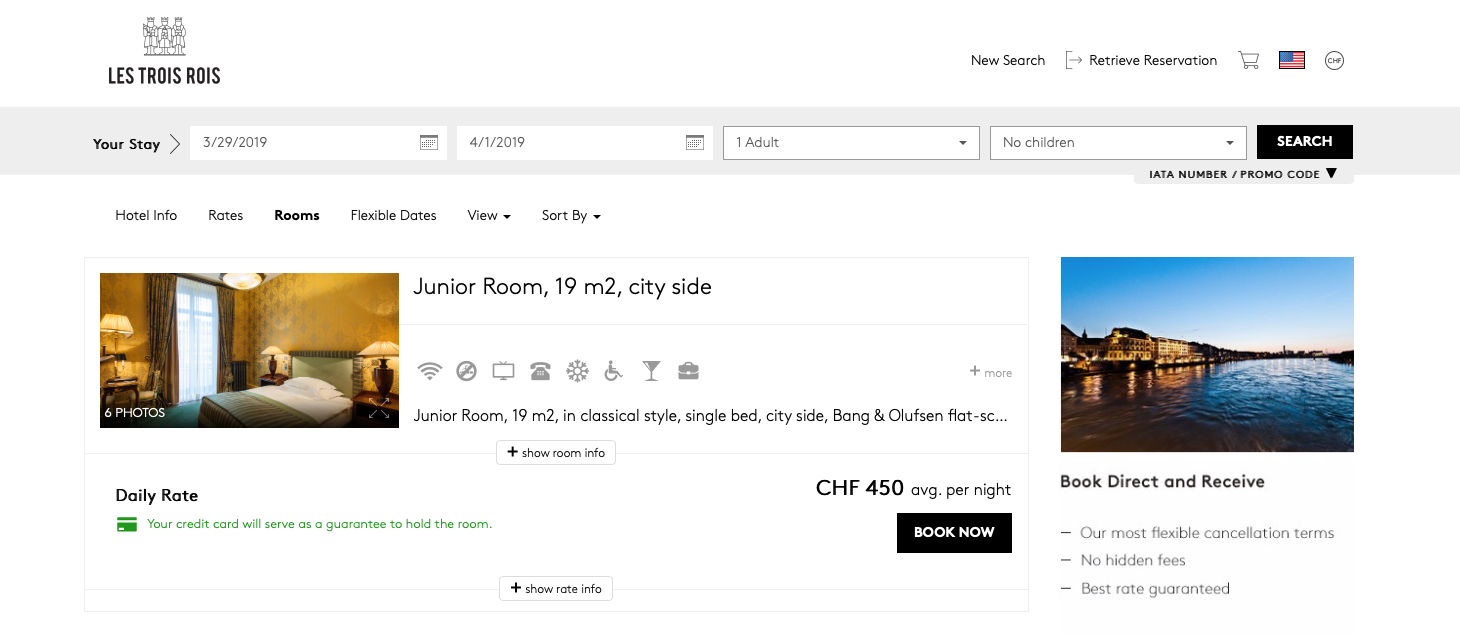The image is a screenshot from a hotel booking website. In the upper left-hand corner, there is a black logo resembling three buildings with the text "Les Trois Rois" written underneath, spelled out as L-E-S T-R-O-I-S R-O-I-S. Adjacent to this on the right-hand side of the page, the words "New Search" and "Retrieve Reservation" appear in black, followed by a card icon, a small American flag icon, and a white circle rimmed in black.

Beneath this header, there is a thick gray bar about an inch wide. On the left side of this bar, the text "Your Story" is displayed in black with a small gray arrow pointing to the right. Next to this are three white input boxes. The first box contains the date "3-29-2019" with a black calendar icon on its right. The second box shows "4-1-2019," again with a black calendar icon on the right. The third box displays "1 Adult" with no children, while a black bar reading "Search" is positioned to the right of these boxes. Below the search bar, the text "beta number/promo code" is displayed in black.

Underneath, several navigation options are listed from left to right: "Hotel Info," "Rates," "Room," "Flexible Dates," "View," and "Sort By."

On the left-hand side is a picture of a hotel room featuring yellow wallpaper, brown curtains, a bed with a padded headboard, white sheets, and a green blanket. To the right of the image, the text "Junior Room, 19 M², Cityside" is displayed in black. Below this is a series of icons: Wi-Fi symbol, a no-smoking sign, a TV, a phone, a circular icon, a handicap symbol, a martini glass, and a shopping bag. Following the icons, the description reads: "Junior Room, 19 M², classical style, single bed, Cityside."

On the right-hand side, the text "Daily Rate" in black is shown above a green credit card icon. Below this icon, the green text states "your credit card will serve as a guarantee to hold the room." To the right of this text, "CHF 450" and "ABG per night" are displayed in black. Additionally, a black "Book Now" button is present.

Below the booking details is an image of a well-lit hotel next to the water. Underneath the image, the text "Book direct and receive" appears, followed by: "- our most flexible cancellation terms," "- no hidden fees," and "- best rates guaranteed."